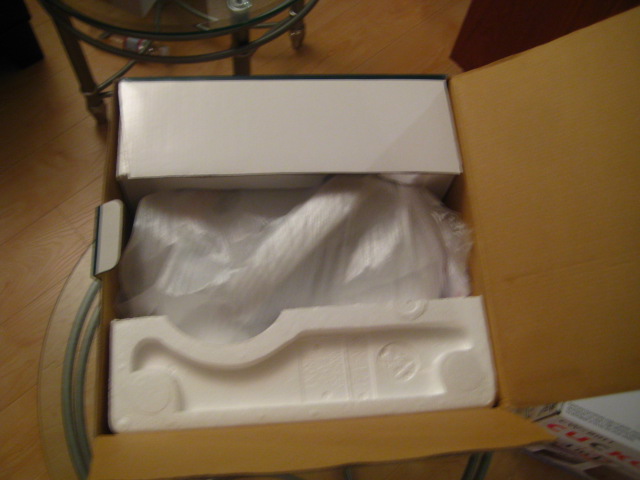In this photograph, we see a large, square cardboard box that has been newly opened and is sitting on a light tan or brown wooden floor. The box contains an unidentified item wrapped in twisted plastic and encased in white styrofoam for protection. One flap of the box is folded over while the other remains closed, and a piece of foam is visible on the side. In the bottom right corner of the photo, another box with partially visible text, showing the letters "CU," "C," and "K," is noticeable. A glass-top table stands in the background, partially obscured, with only three of its legs visible. The box appears to be situated on a carpet featuring a round gray border. The overall scene suggests the setting is a living room, though most of the background details remain indistinct.